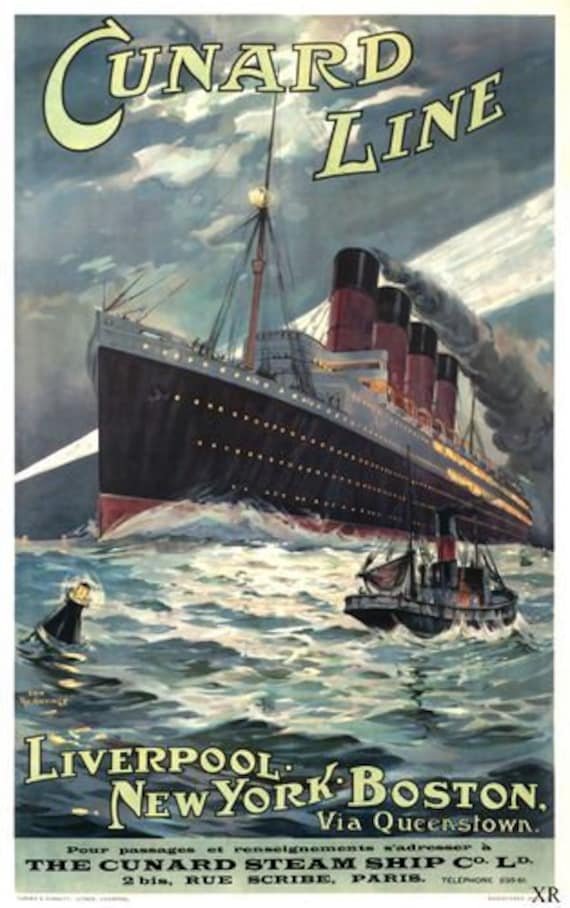This vintage-style poster, possibly from the 1930s, advertises the Cunard Line, spelled C-U-N-A-R-D. Dominating the artwork is an ocean liner, strongly resembling the Titanic or the Queen Mary, plowing through the Atlantic Ocean. The choppy waters in the foreground suggest rough seas, with waves crashing vigorously against both the large ship and a smaller tugboat nearby. Adding to the drama is a buoy with a light at the top, seen rocking violently in the ship’s wake. The lower portion of the poster displays destinations: "Liverpool, New York, Boston, via Queenstown," along with some French text that, though partially blurry, reads "Pour Passagers" and references the Cunard Steamship Co. Ltd. The intricate artwork and its pastel hues evoke a nostalgic and old-fashioned aesthetic, accentuating the grandeur and historical significance of this maritime voyage.